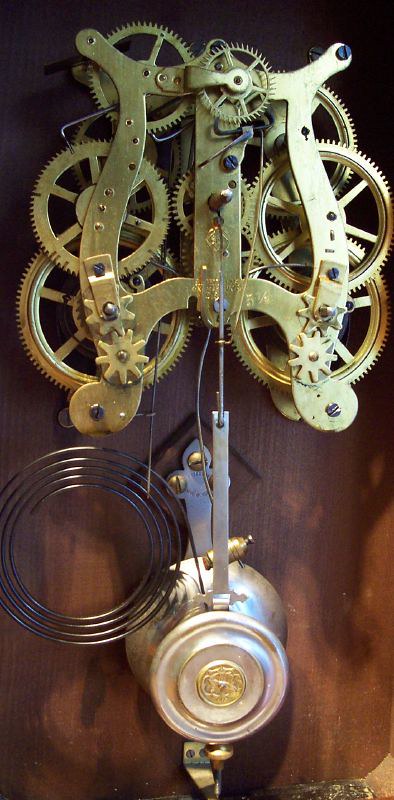The image depicts a highly intricate mechanical device, set against a weathered wooden background. At the forefront of the image is a glass screen, offering a protective barrier for the delicate inner components. On the left side, there are four different types of circles, each featuring an opening in the center, with the smallest circle being particularly prominent. 

Towards the bottom of the mechanism, a metallic knob, resembling a doorknob, is designed to spin, indicating its functional role. Above it lies a complex assembly held together by metal construction, showcasing a total of ten interlocking gears. In addition to these primary gears, there are four smaller, pinwheel-like gears visible from the front, contributing to the overall complexity. 

The image likely reveals the internal workings of a sophisticated device, suggesting that it has been opened up to display its intricate mechanical structure.